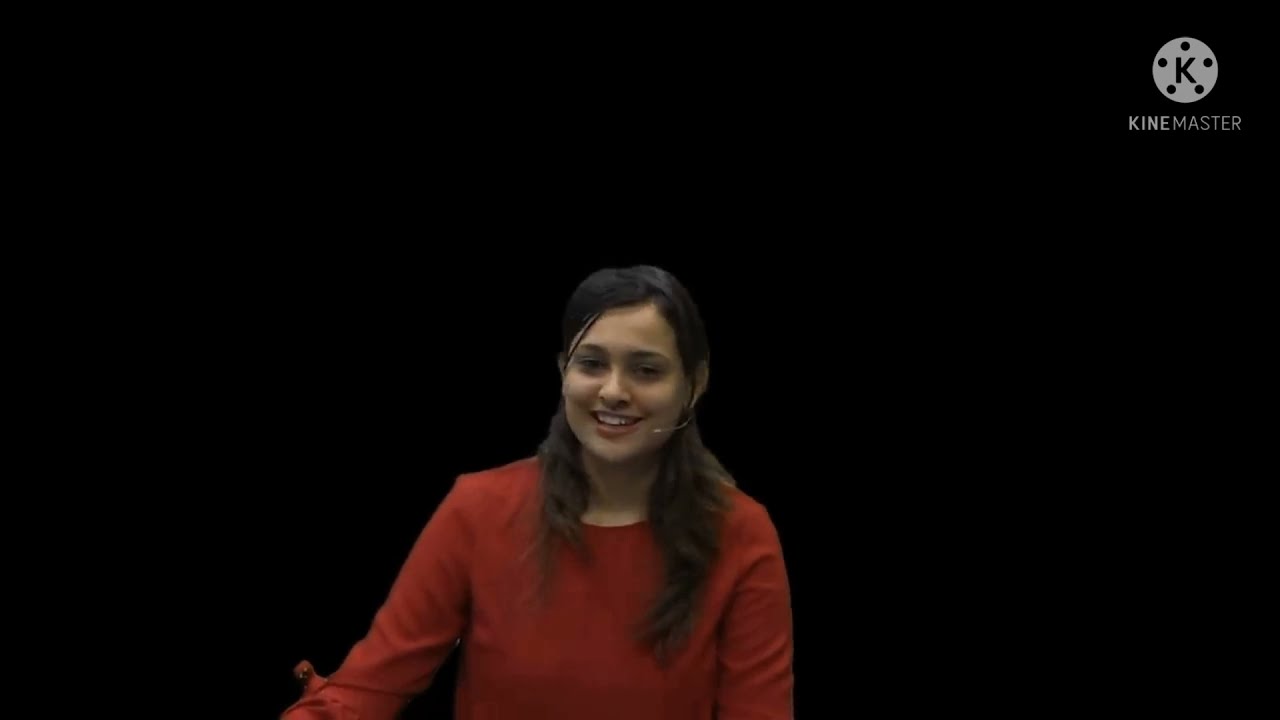The image features a young Hispanic girl with a big smile on her face, revealing her teeth with her mouth open. She has long black hair pulled back behind her head, with a single strand falling down the left side of her face, and the rest cascading over her shoulders and chest. The girl is wearing a long sleeve orange dress and has a thin microphone extending from her left ear towards her mouth. She stands slightly off-center towards the left, and her head is tilted slightly to the left. The background is completely black, creating a stark contrast that highlights her features. Positioned in the top right corner is a gray circle with five dots surrounding the letter "K" in the center, accompanied by the text "KineMaster" in gray underneath, suggesting the logo of the KineMaster software. The overall setting suggests that this might be a screenshot from a presentation she is giving, inferred by the presence of the hands-free microphone.